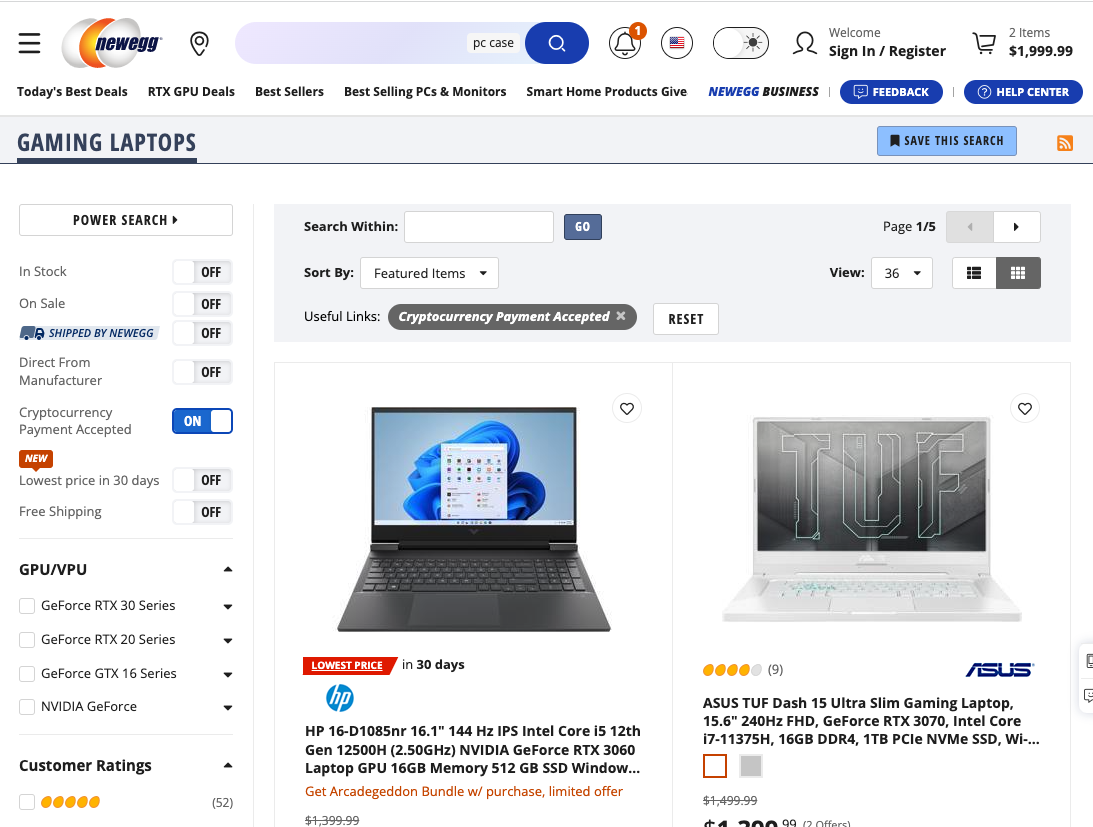This webpage from the Newegg website prominently features the Newegg name and logo at the top left. The main body of this page has a white background, with various images and text scattered throughout. Centered on the left side is an opened laptop displaying a Windows desktop. Directly below the laptop, a red rectangular box announces "Lowest price in 30 days," with the HP logo positioned beneath it. To the right of this laptop, an ASUS TUF-15 Ultra Slim Gaming Laptop is showcased, with the ASUS logo displayed at the bottom right of the laptop image. 

At the very top of the page, there is a user-friendly search bar that is shaded light purple, complemented by a dark blue search button adorned with a magnifying glass icon. The search term "PC case" has been entered into this search bar. Adjacent to the search bar on the right, an alarm bell icon with an orange circle containing the number "1" signals a new message. Further to the right, an American flag is visible, indicating the regional settings of the website.